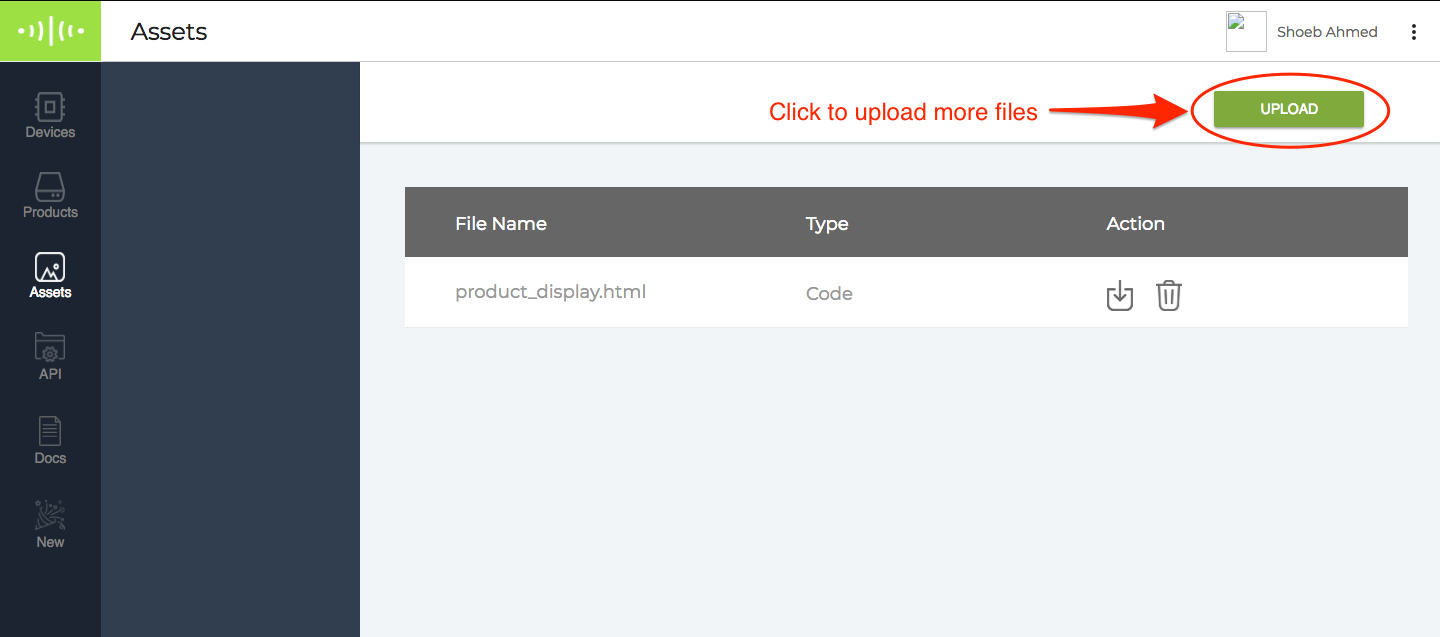The interface of the website features several distinct sections and elements which help in navigating and managing assets. On the top left-hand corner, there is a small green box adorned with white lines. Adjacent to this is the word "Asset" written in black, set against a white background. Positioned on the top right-hand side is the user's name, "Shoeb Ahmed," formatted with the first name "S-H-O-E-B" and the last name "A-H-M-E-D." Below this, a thin gray line stretches horizontally across the screen.

On the left-hand side, a navy blue rectangle houses multiple tabs including "Devices," "Products," and prominently in bold white text, "Assets," indicating the current selection. Other tabs labeled "API," "Docs," and "New" are also present within the same section.

Directly across from the navigation tabs, on a white background, a red message prompts the user with "Click to upload more files," accompanied by a red arrow pointing towards an oval shape. Inside this oval is a green box that contains the word "Upload" in white font.

Beneath this white section, the backdrop transitions to a light gray. Within this area, two main rectangles are distinct. The first is dark gray and contains headings starting from the left: "File Name," "Type," and "Action," all in white text. The subsequent white rectangle features an entry in gray text that reads "product_display.html," followed by "code," an icon of a trash can, and a downwards arrow.